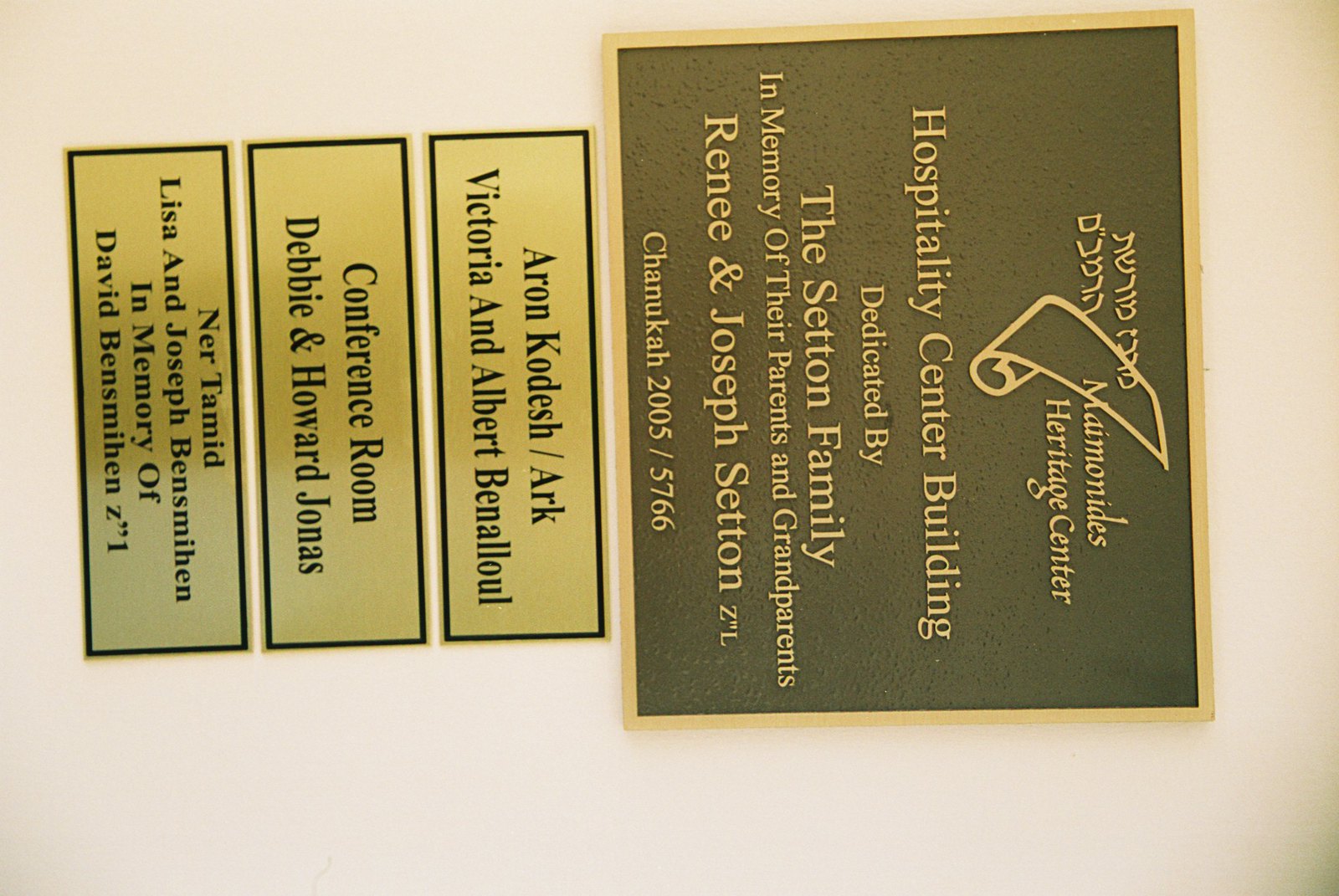The photograph, which is currently oriented incorrectly in landscape, should be rotated 90 degrees counterclockwise for proper viewing. At the top of this portrait-oriented image is a large black plaque with a gold border. In the top left corner of the plaque, there is Hebrew writing, while the top right corner features a gold-outlined scroll logo next to the text "MAIMONIDES Heritage Centre." The plaque reads: "Hospitality Centre Building, dedicated by the Seton family in memory of their parents and grandparents, Rene and Joseph Seton, Hanukkah 2005, 5766." Below this central plaque are three smaller plaques, aligned vertically. Each of these plaques has a gold background with black text and black outlines. These are dedication plaques with various names listed: the "Aaron Kodesh Ark, Victoria and Albert Benalaw," the "Conference Room, Debbie and Howard Jonas," and the "Ner Tamid, Lisa and Joseph Bensmithen, in memory of David Bensmithen."